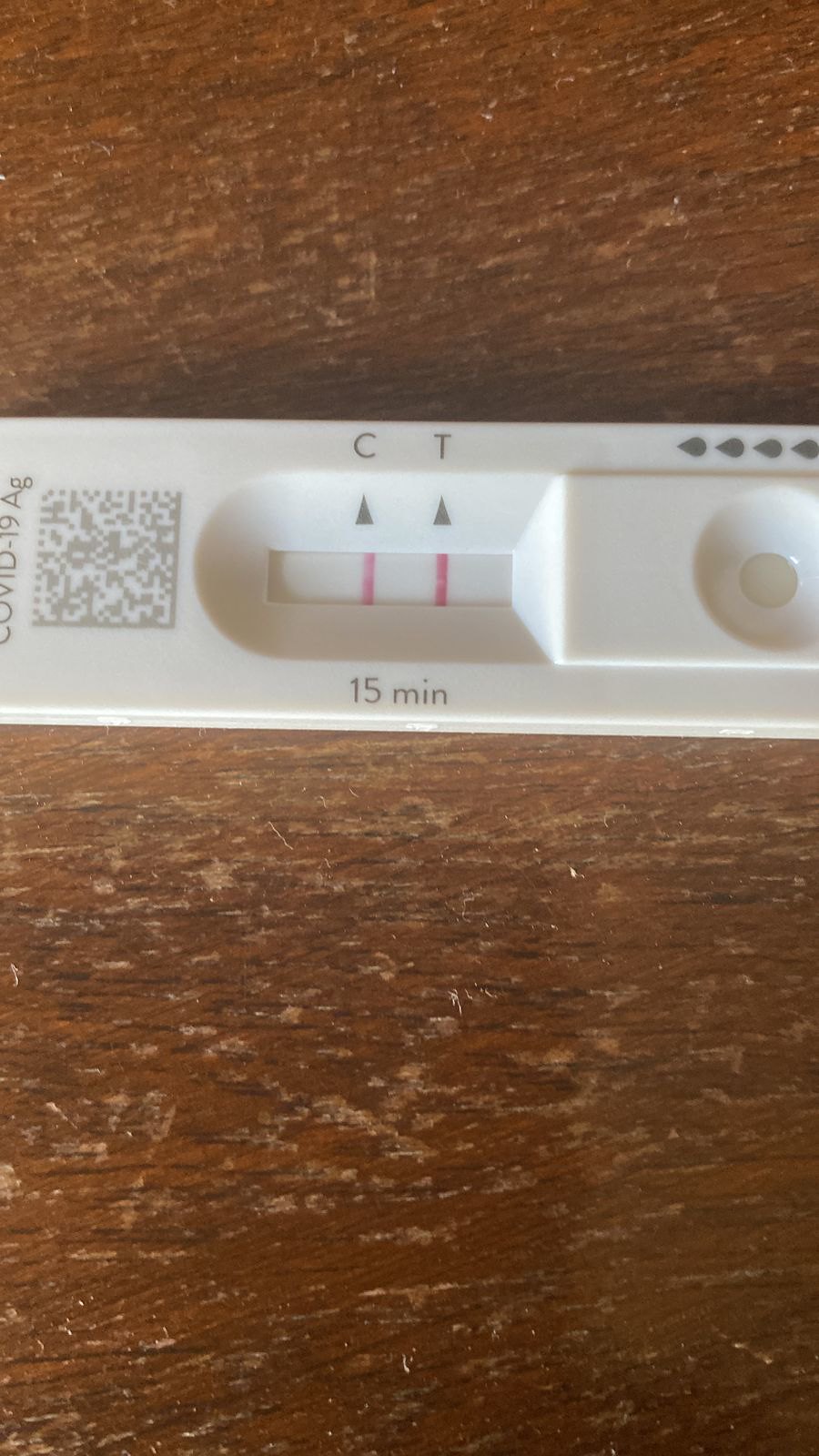This image showcases an at-home COVID-19 test prominently displayed across the entire width of the picture. The test, which is white and rectangular, sits on what appears to be a brown tabletop or shelf. The surface of the tabletop is medium brown with a mix of lighter brown specks and darker wood grain lines, offering a textured background.

The test itself is partially visible, focusing primarily on the section that indicates the test results. At the top of the visible section, "COVID-19 AG" is printed, followed by a light gray QR code. Below the QR code, there is an arch-shaped depression containing the result display window.

In the display window, there are two red lines indicating the test result. The left red line is positioned under a triangle pointing upwards to a capital "C," while the right red line is situated under a similar triangle pointing to a capital "T." Below these lines, the text "15 MIN" is visible. The format of the test then returns to its standard rectangular shape.

To the upper right of the test, four gray water droplet icons are seen, situated above a circular depression. These elements are part of the overall design and markings of the at-home COVID-19 test.